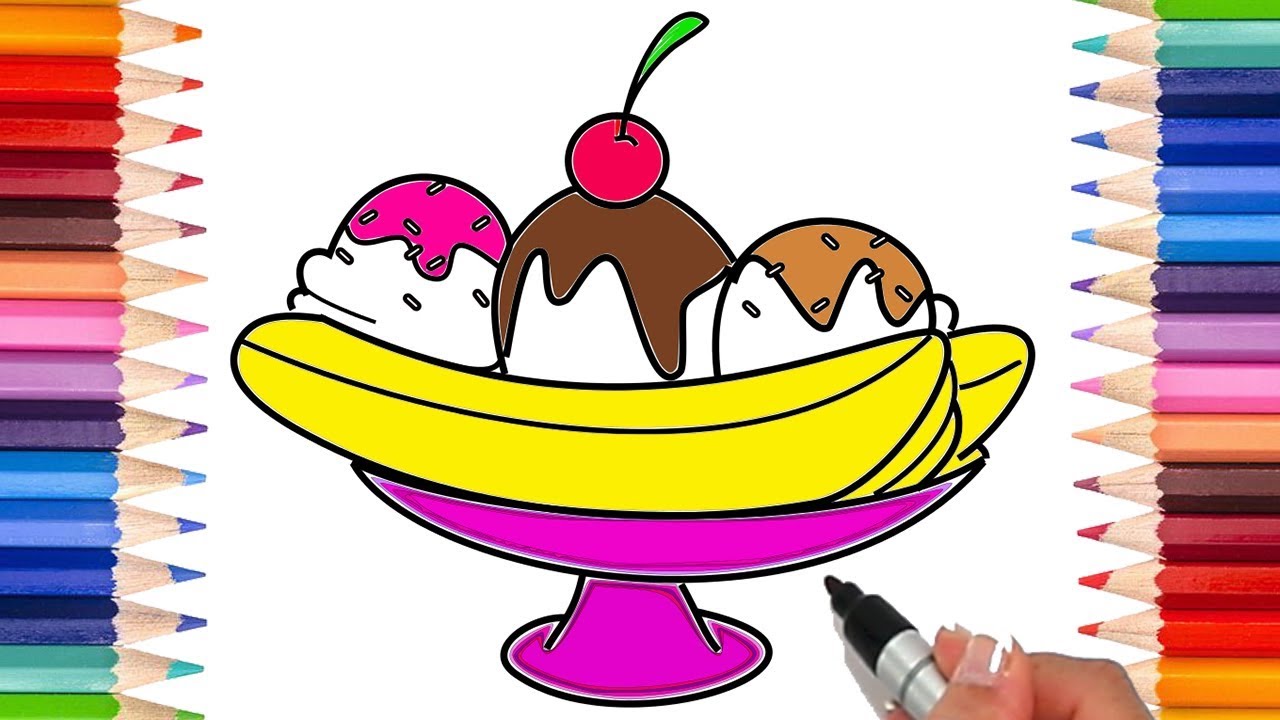The image captures a vibrant and detailed scene of a meticulously drawn illustration of a banana split sundae nestled in a magenta bowl. Surrounding the sundae are an array of sharpened colored pencils arranged in a rainbow spectrum on both the left and right sides of the image. The sundae features three distinct scoops of ice cream: the left scoop is adorned with white sprinkles and magenta syrup, the middle scoop is drizzled with chocolate syrup and topped with a cherry, and the right scoop is embellished with caramel syrup and white sprinkles. Anchoring the bottom right corner of the image, a manicured hand with a French manicure holds a black permanent marker, giving the impression that the drawing is in progress or newly completed. Despite the hand-drawn appearance, the graphic quality of the illustration suggests it may have been enhanced or created digitally.